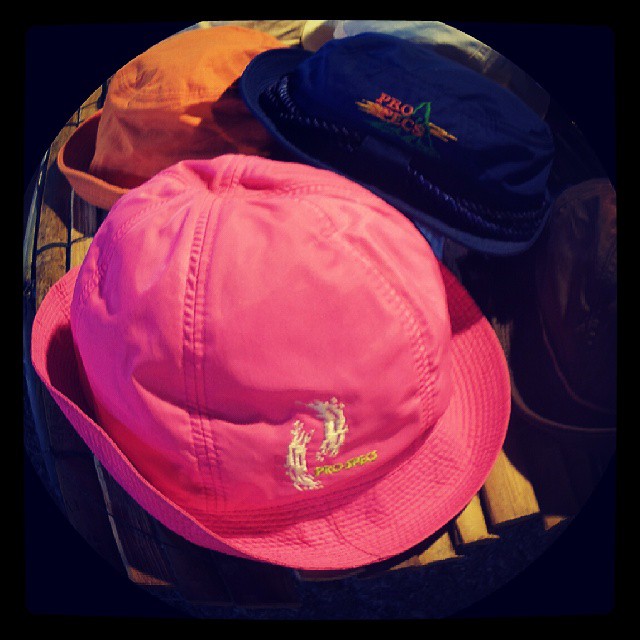In this image, a striking array of colorful hats is presented against a stark black background, making the vibrant colors pop vividly. At the forefront is a bright pink hat labeled "Prospect Hats" in bold yellow writing, resembling a bucket hat. Positioned behind it is a navy blue hat with similar "Prospect Hats" text in contrasting orange, adorned with a fisherman's rope detail, suggesting a fishing hat style. Further back, an orange hat of the same style is partially visible. Also, to the right side, there seems to be a brown hat, slightly obscured by shadow but maintaining the bucket style seen in the others. All these hats are displayed on a wooden surface, giving the setup a rustic feel. The slight fisheye lens effect accentuates the hats' colorful and playful nature, drawing immediate attention to the central pink hat while subtly unveiling the variety and details of those behind it.